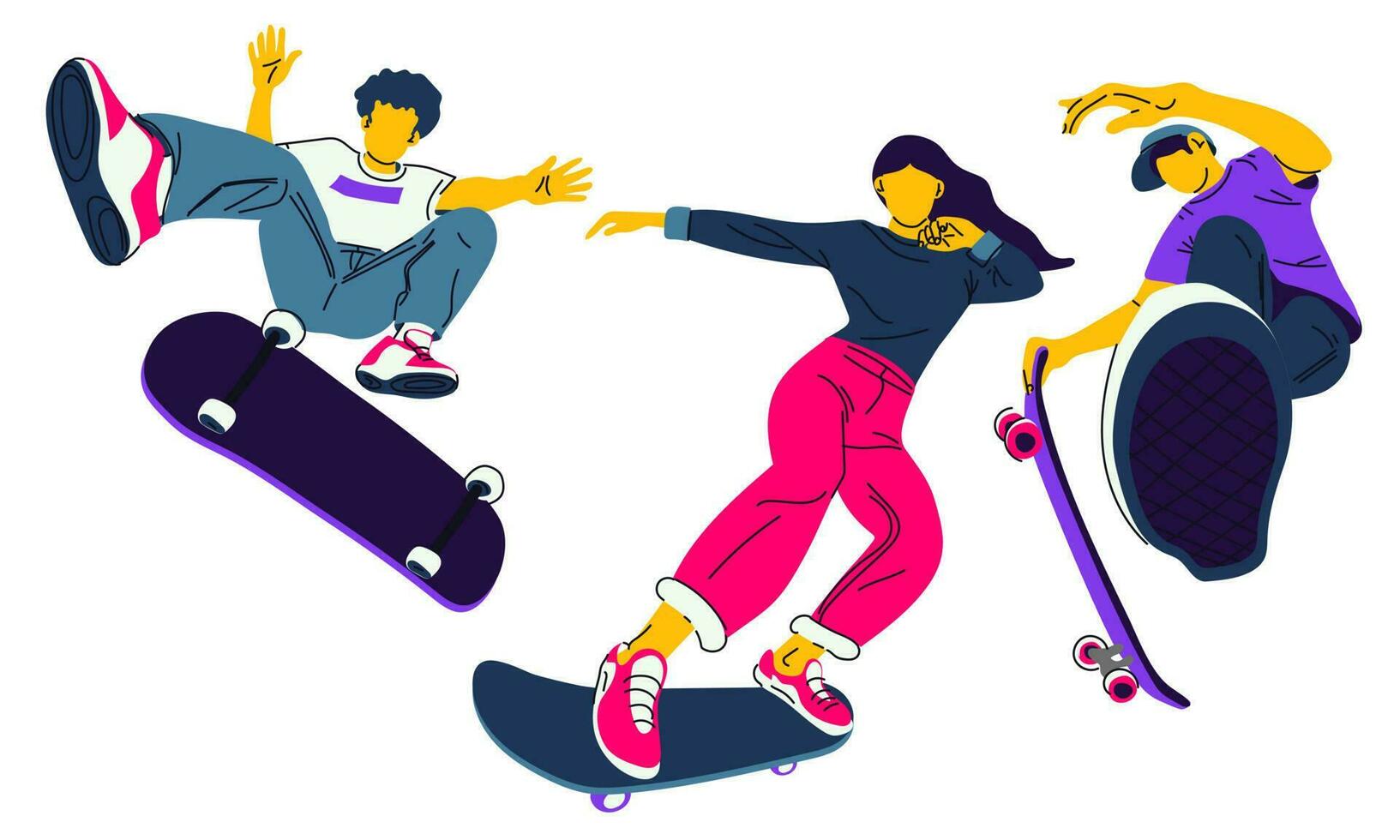In this vibrant cartoon-style drawing, the image captures three skateboarders in mid-action, vividly showcasing their dynamic tricks and colorful attire. On the left, a boy with yellow skin and dark black hair is flipping his skateboard. He wears blue jeans, white sneakers with pink trim, and a white short-sleeved shirt with a purple logo. His skateboard is purple with white wheels. In the center, a girl with long flowing black hair is riding her blue skateboard with purple wheels. She dons pink cuffed pants, pink sneakers, and a long blue sleeve shirt. Her right arm extends outward as she maintains her balance. To her right, another boy, also with yellow skin, is holding onto his purple skateboard with pink wheels while performing a trick. He sports a green baseball cap, a purple shirt, blue sneakers, and blue jeans. All three characters have a faceless design, adding a unique artistic touch to the energetic scene.